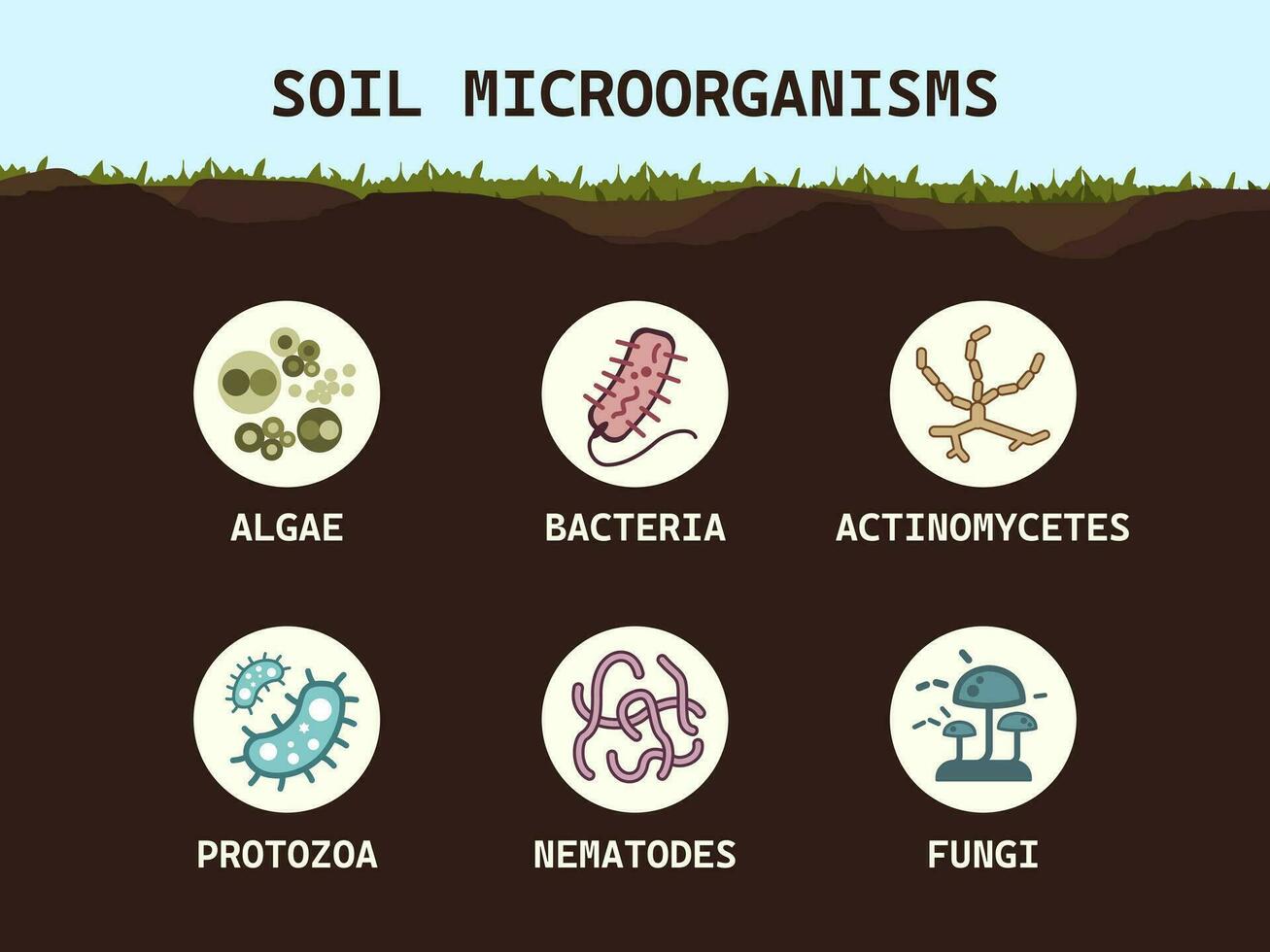This detailed infographic illustrates soil microorganisms in a rectangular image wider than it is tall. The top fifth of the image features a cyan sky, and just below it is a thin layer of green grass. Beneath the grass, a deep brown soil layer with slight color variations occupies the remaining four-fifths of the image. Six cream-colored circles are arranged in two rows within the soil, each containing a computer-generated depiction of a specific microorganism, along with its name in white text. 

The microorganisms are depicted as follows, from left to right, top to bottom: 
1. Algae: illustrated as various shades of green circles.
2. Bacteria: depicted as a maroon shape with an elongated tail and interior squiggly lines.
3. Actinomycetes: shown as a brown tree-branch-like structure.
4. Protozoa: resembling two kidney beans with cyan lines and white circles within a cyan interior.
5. Nematodes: illustrated as pink squiggly lines.
6. Fungi: depicted as three blue mushrooms with lines radiating from one side.

The infographic is titled "Soil Microorganisms" in black letters above the grass, capturing the intricate ecosystem beneath the soil's surface.